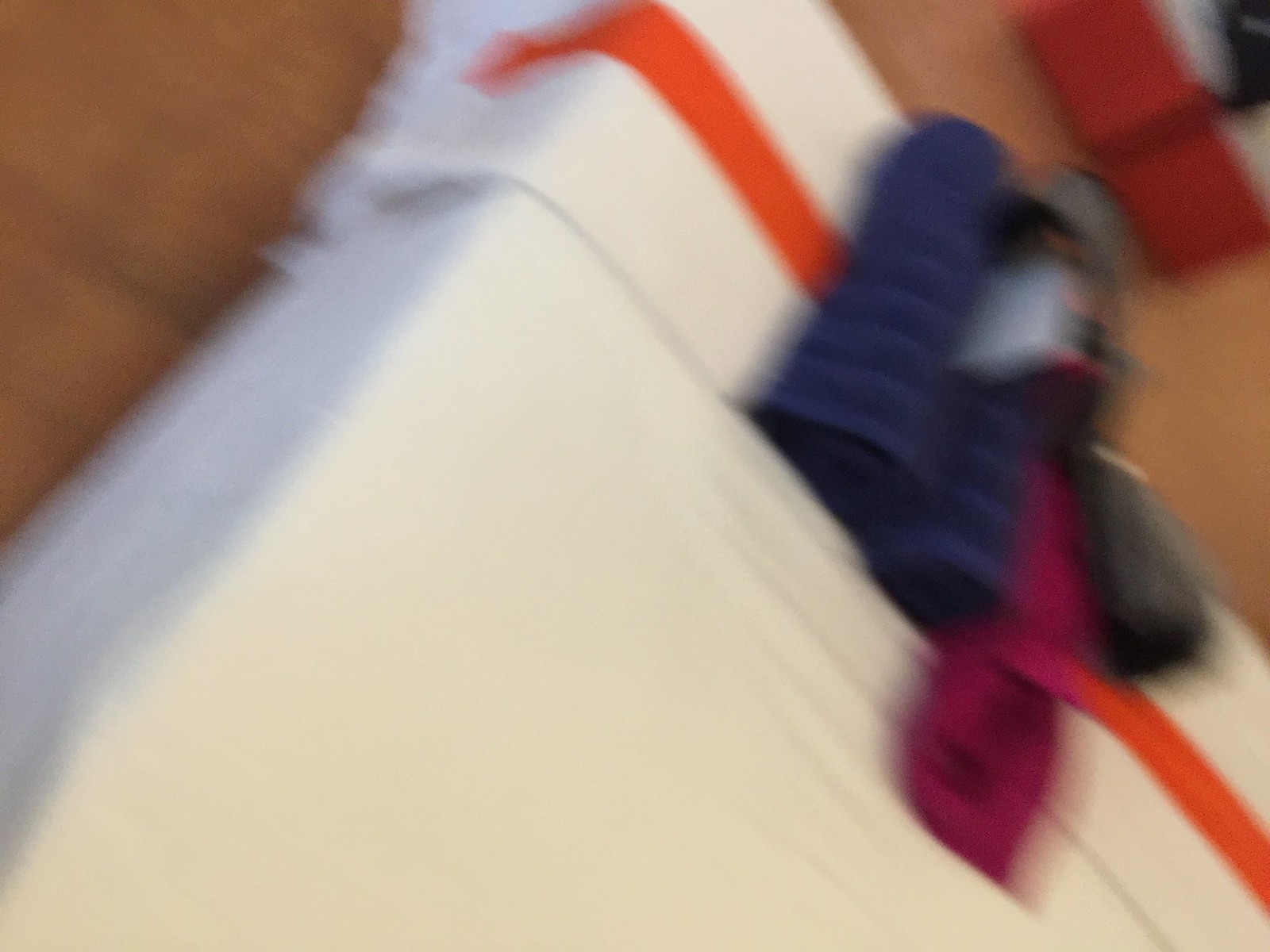A blurry, top-down photo captures an off-angle view of what appears to be the top left corner of a bed. The bed is covered in white bedding with a prominent orange stripe running across the top edge. Placed in the middle of the bed are two rolled-up, dark blueish-purple objects, possibly towels, positioned side-by-side. To the right of these objects lies a pinkish-magentas cloth and something black running next to it. A rectangular lighter object is located between the two rolled-up blue items. The bed itself seems low to the floor, which is a beige or orangish color. Further back, nearer the foot of the bed and still within the frame, some orange and white rectangular items are visible, possibly boxes, along with what could be a quilted jacket and perhaps a sweater in a deep fuchsia or magenta shade. The entire image is grainy and blurred, making the exact details hard to distinguish.